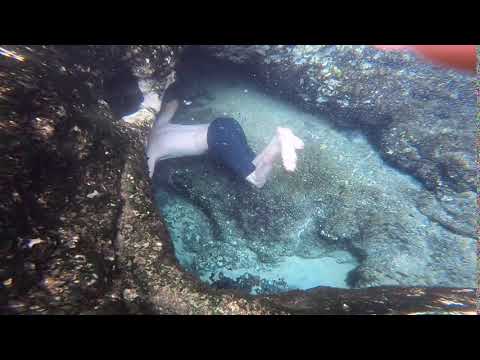The image depicts a vivid underwater scene with a snorkeler in blue swim trunks partially submerged in crystal-clear, teal-blue water. They are entering a rocky underwater cavern, with the head of the snorkeler already inside the cave while the rest of their body remains visible. The surrounding environment features rugged, brown rock formations with patches of algae and small shells scattered across the surface. The water is strikingly clear, giving a pristine view of the scene. The top and bottom of the image are framed by black horizontal bars, emphasizing the landscape with its diverse colors, including shades of blue, green, brown, white, and hints of red in the upper left corner. Overall, the image captures the serene yet adventurous moment of a snorkeler exploring an underwater cavern amidst a richly textured rocky landscape.